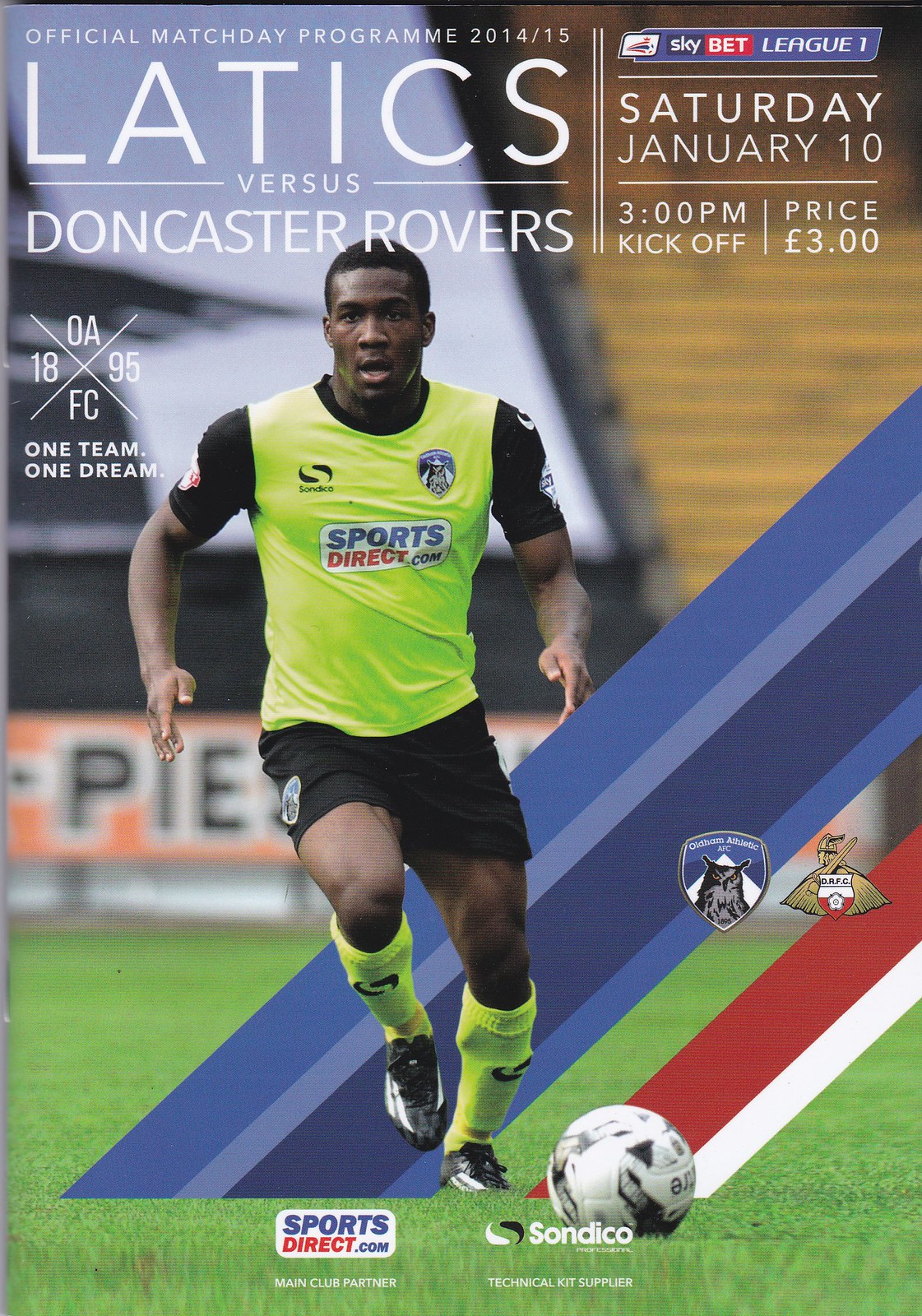The front cover of this football program for the Latics versus Doncaster Rovers features a dynamic action shot of a black footballer in the midst of play, intensely focused on a ball in front of him. He is sporting a neon green jersey with black sleeves, paired with black shorts, neon green socks, and black sneakers. Adorned on his jersey are the logos of sportsdirect.com and another logo with an 'S'. Superimposed over the background, there are diagonal blue and gray bars running from the bottom left to the top right, as well as a blue and white band which includes the team emblems: a Viking with a helmet and sword for Doncaster Rovers, and an owl on a blue background for the Latics. The top of the cover reads, "Official Match Day Program 2014/15 - Latics versus Doncaster Rovers," with the details "Saturday, January 10th, 3 p.m. kickoff," priced at £3. The left side features the slogan "OA 1895 FC, One Team, One Dream," while the right side shows sponsors such as sportsdirect.com and Sandico. Behind the player, a slightly blurry green field and empty stands with advertisements, including one that reads 'pie,' complete the vivid scene.